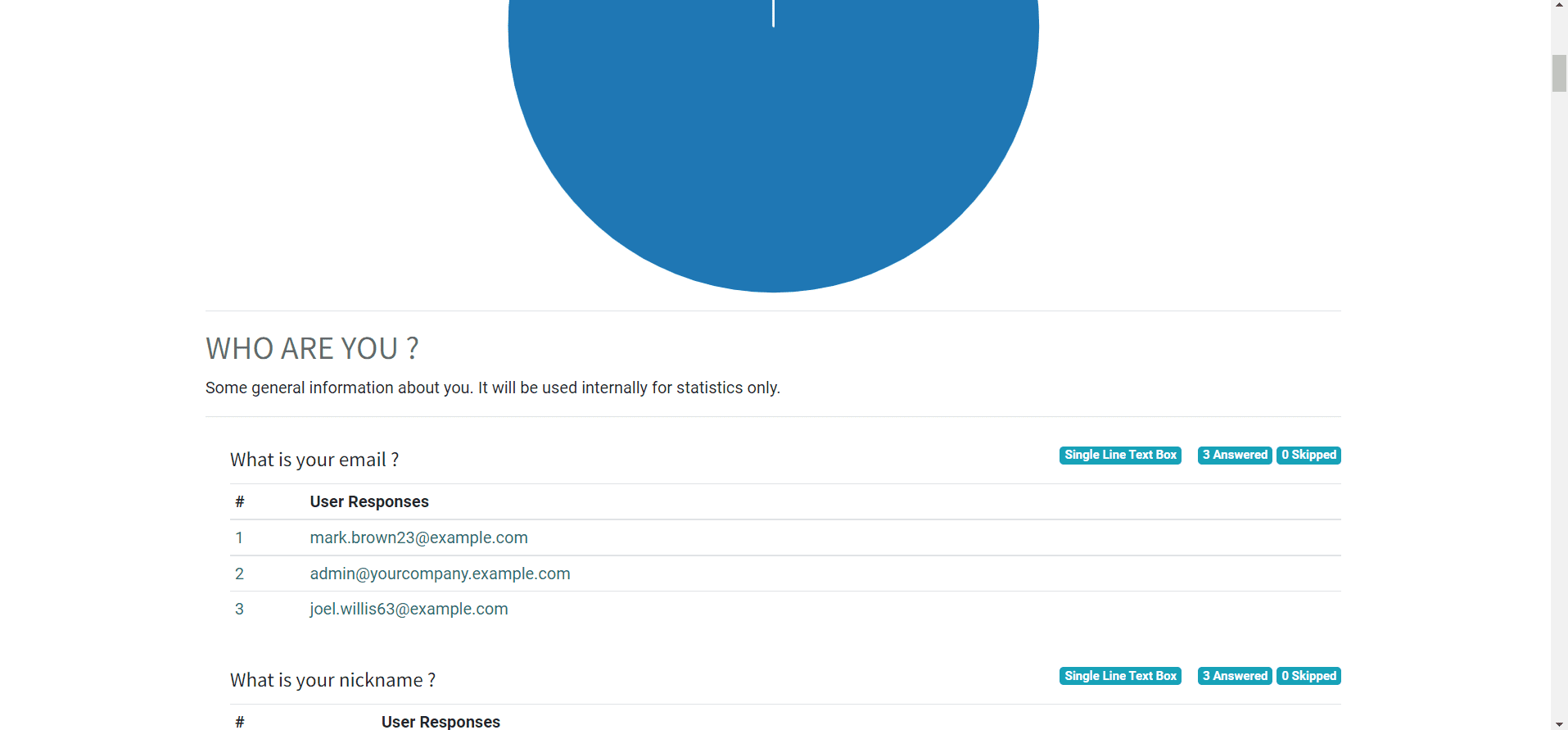At the top center of the page, a partially visible pie graph is displayed against a medium blue background. A thin white line descends from the top center of the graph, leading to a faint gray divider line below. On the left side, the text "WHO ARE YOU" appears in capital gray font with a small black question mark spaced underneath. Below this, a brief description reads, "Some general information about you. It will be used internally for statistics only." A second divider is present underneath.

Further down, "WHAT IS YOUR EMAIL?" is written in gray on the left, followed by another divider. To the left in black, a bold hashtag symbol indicates the section "USER RESPONSES" in bold black lettering. A divider line follows, then a blue number "1" introduces a listed email: mark.brown23@example.com. Another divider separates this entry from the next: blue "2" and admin@yourcompany.example.com. Additional dividers structure the following email, blue "3", reading joel.willis63@example.com. 

Subsequently, "WHAT IS YOUR NICKNAME?" is positioned with a space and a question mark. To the left, another bold black hashtag is tagged with the text "USER RESPONSES" in bold black lettering.

Towards the top right of this section, three thin rectangular boxes with a teal background appear, each containing small, bold white text. The first box reads "Single line text box," the second "3 answered," and the third "0 skipped." Identical boxes appear near the "WHAT IS YOUR EMAIL?" header at the page's top.